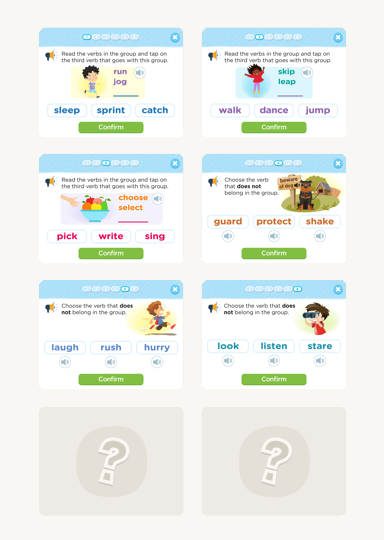The screenshot captures a digital interface set against a pale, very light green background. This interface features six distinct images, arranged neatly in two columns. Each image is framed with a light blue strip across the top.

- The first image in the upper left highlights a cartoon character actively running and jogging. Beneath this character, the words "sleep, sprint, catch" are displayed in blue text. Directly below this, a green button labeled "confirm" in white text is visible.
  
- The second image, situated in the upper right, depicts a cartoon character dressed in a red dress. Below this character, the words "walk, dance, jump" are elegantly scripted in blue.

The remaining four images continue in a similar format, each portraying different activities undertaken by various cartoon characters. The images in the bottom row, however, are notably grayed out and adorned with question marks, indicating content that is either locked or yet to be revealed.

This detailed compilation not only provides visual engagement with the cartoon characters but also categorizes their activities clearly, enhancing user interaction with the digital platform.